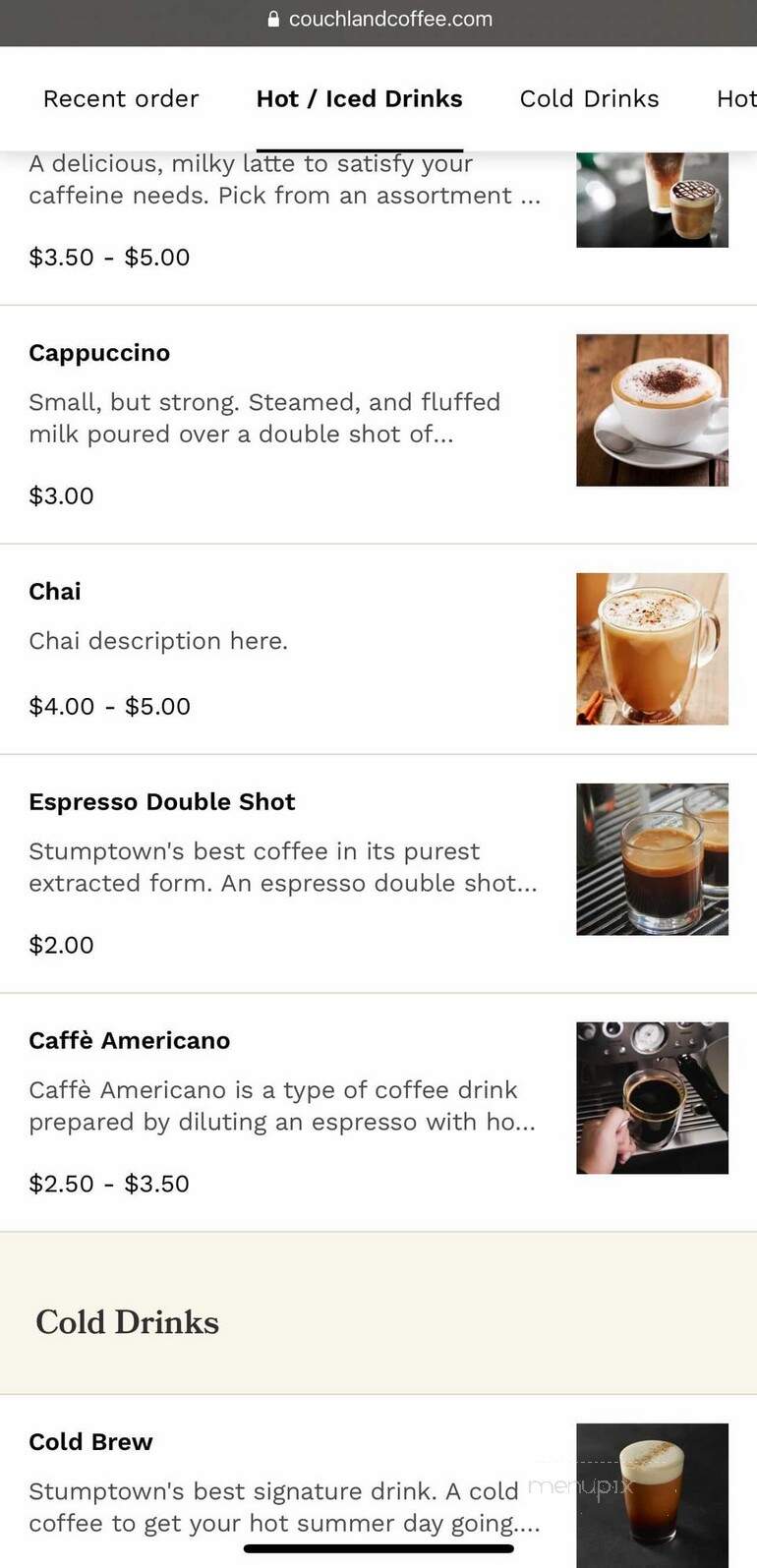A user is browsing the menu of a fancy café website called CouchLandCoffee.com on their phone. The visible sections include "Recent Order," "Hot/Iced Drinks," "Cold Drinks," and possibly more categories as you scroll right. In the "Hot/Iced Drinks" section, options like a latte priced between $3 to $5, a cappuccino for $3, chai for $4 to $5, a double shot of espresso for $2, and a café americano for $2.50 to $3.50 are listed. The "Cold Drinks" category is partially visible, showing "Cold Brew" with the price cut off. The café exudes a professional atmosphere with reasonable prices, indicative of an older menu. Notably, half of the drinks feature intricate foam art, adorned with sprinkles of cinnamon or ginger, enhancing their visual appeal.